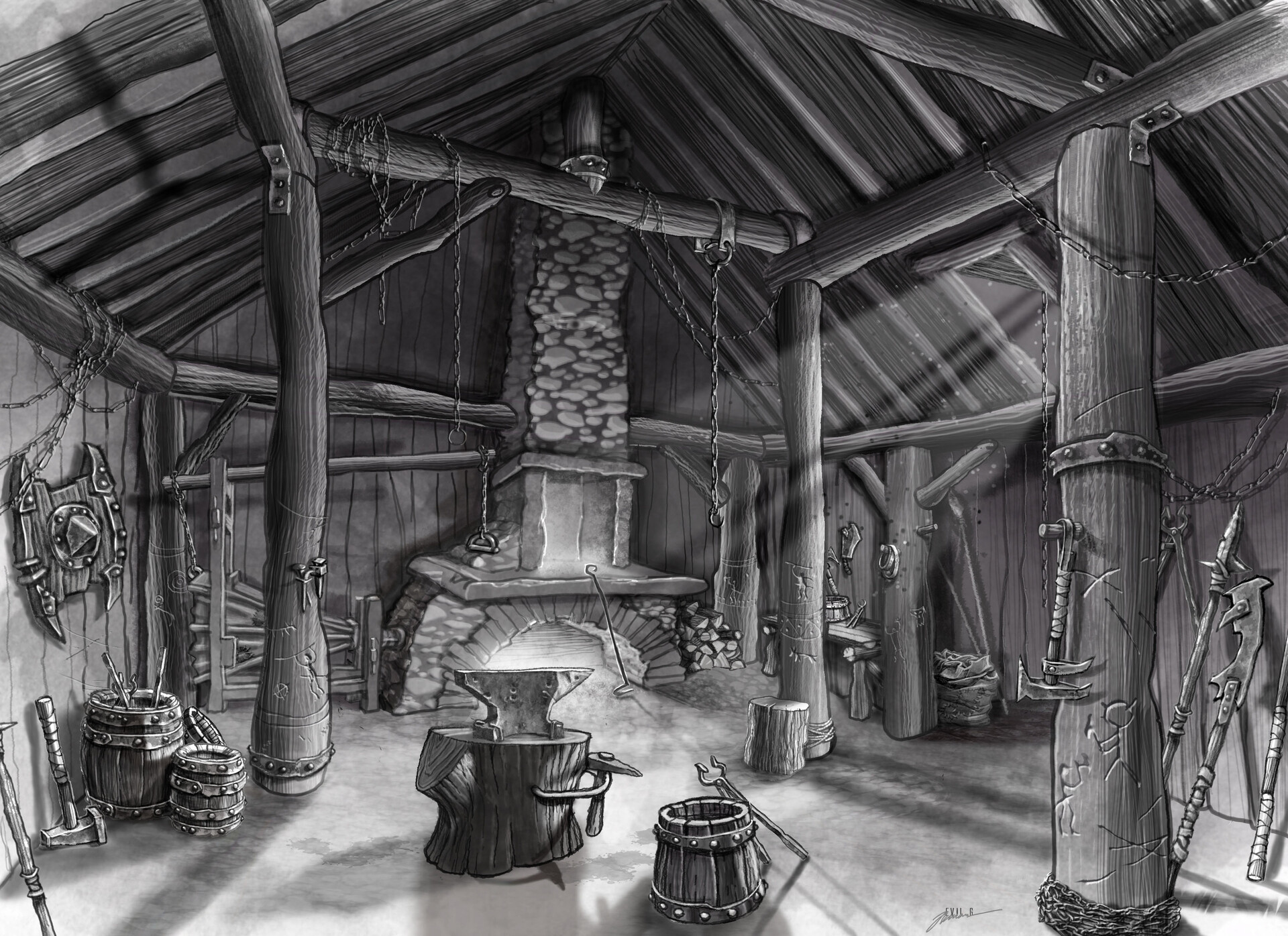This is a highly detailed black and white drawing depicting the interior of an old cottage, which appears to function as a blacksmith's workshop. The centerpiece of the room is a large stone furnace, possibly with a fire burning within, though it's somewhat obscured by the structure. Supporting the wooden ceiling are various tree trunks used as columns, some of which are attached by bolts. Chains hang from the rafters, adding to the authenticity of the scene.

The cottage is filled with various pieces of equipment and metal tools, including an anvil set on a tree trunk, hammers, swords propped against the walls, and sharp tools. Barrels scattered throughout the room seem to store additional tools and metalwork items. A simple lattice of wooden boards helps uphold the wooden ceiling. One wall prominently features a battle shield, suggesting readiness for combat or trade. The meticulous illustration implies an active workspace, even in the absence of any human presence, creating a vivid sense of an industrious, lived-in environment.